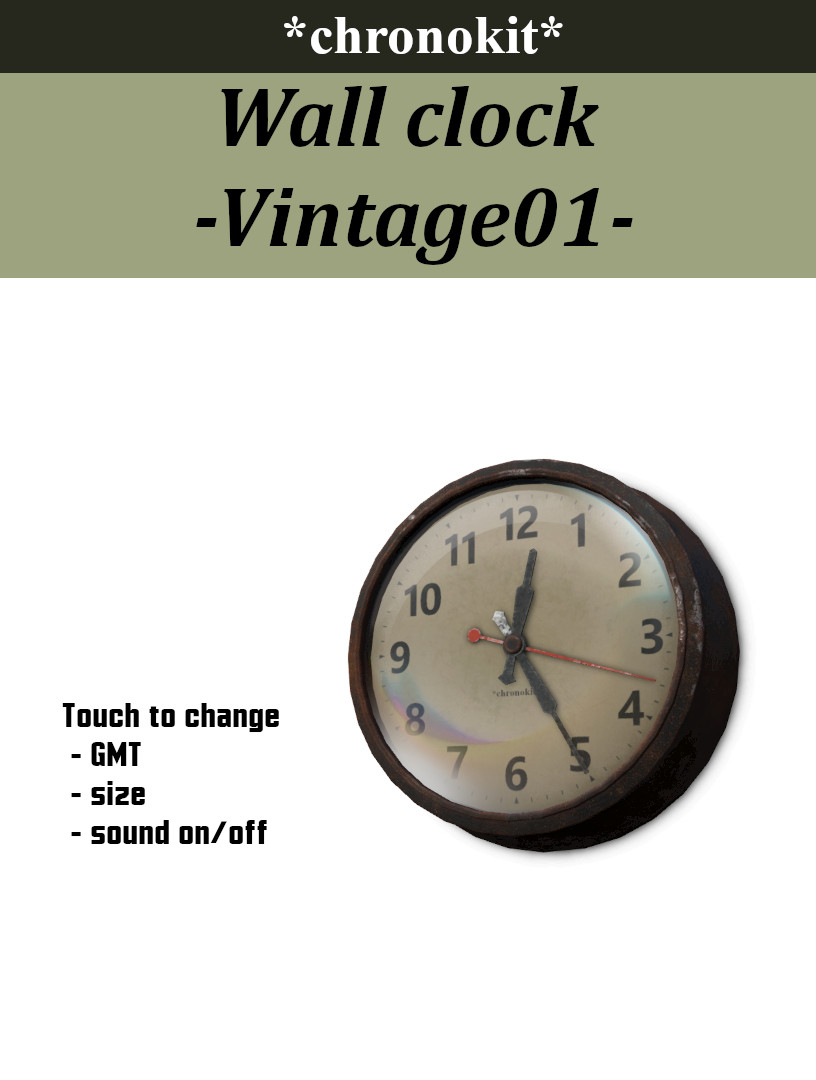The image showcases a vintage wall clock with a white face and black numerals. The clock has a black edge and black hour and minute hands, complemented by a striking red second hand. Above the clock, there is a black banner with white letters reading "Chrono Kit." Below the banner, the light gray background displays additional text in black letters: "Wall Clock" and "Vintage 01." To the left of the clock, the text "Touch to Change" appears, followed by options: "GMT," "Size," "Sound On," and "Sound Off." The current time on the clock is set to 12:25.